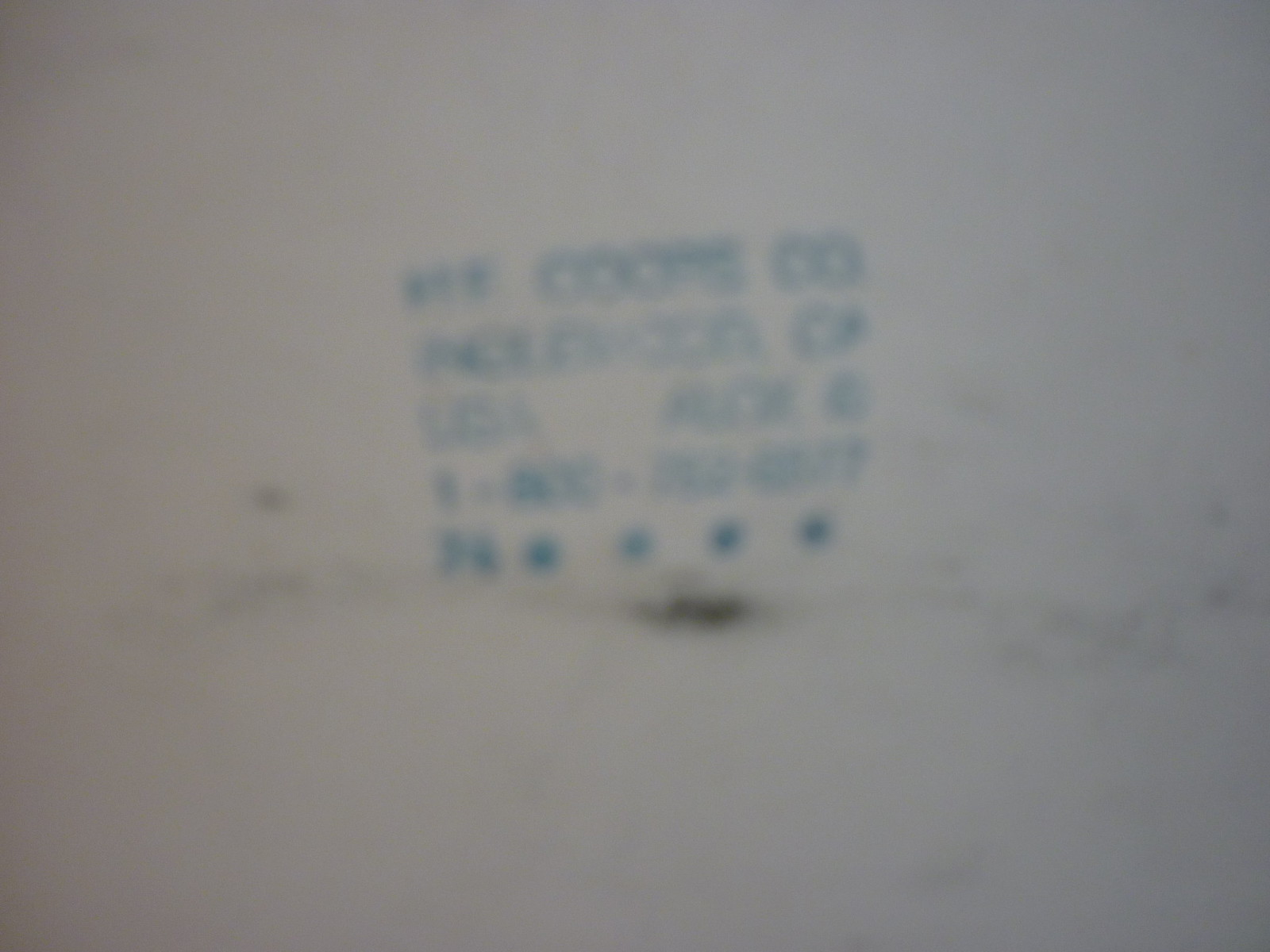The photograph captures a pale lilac-gray background with a series of blue writings that are mostly illegible. At the top, there are two smudged letters followed by a space and then "C-O-O" with possibly more characters after another space. The line below begins with "P-O" followed by an unreadable sequence with intermittent spaces and letters. The third line clearly spells out "USA" with spaces on either side, but the surrounding letters are difficult to decipher. Below this, another line contains a partially visible word ending in "X," suggesting it could be related to a size indication, though the characters to the right remain unclear. The final line on the left side features a set of four distinct blue dots. Beneath this, a noticeable black smudge and additional dark markings, resembling pencil smearings, are visible, extending to the right and slightly downward from the text.